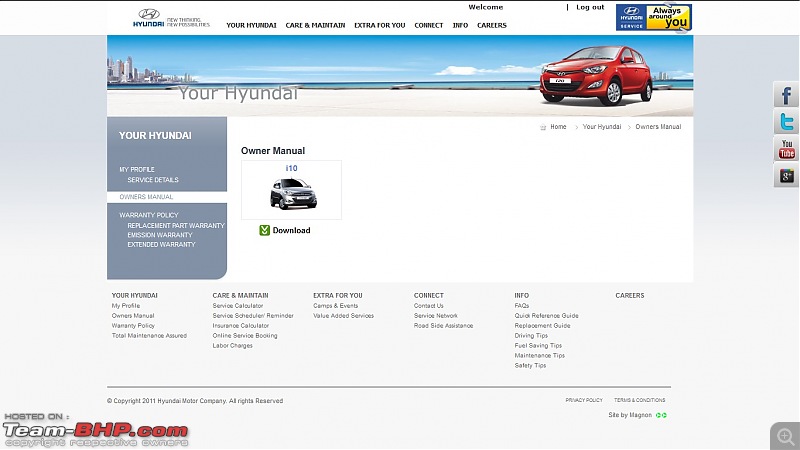This image showcases the user interface of the Hyundai website. At the very top of the image, a thin black line spans the width of the screen. Beneath this line, the Hyundai logo and name are positioned to the left. Along the top of the screen, a white navigation bar features several menu options in black text: "Your Hyundai," "Care and Maintain," "Extra for You," "Connect," "Info," and "Careers." To the right of these options, there is a logout link and the Hyundai icon in dark blue, accompanied by the slogan "Always Around You" inside a yellow rectangle background.

In the central section of the page, a prominent banner runs nearly across the entire width of the screen, displaying the text "Your Hyundai" next to an image of a red Hyundai car. Below this banner, the main content area of the website is visible. It includes a section titled "Your Hyundai in My Profile," presented against a gray background on both sides. This section features options for Service Details, Owner Manual, Warranty Policy, Replacement Part Warranty, Extended Warranty, and Emission Warranty—where the "Owner's Manual" is currently selected and available for download on the right.

At the bottom of the page, additional menu options are available for user interaction, enhancing the navigational experience within the Hyundai website.